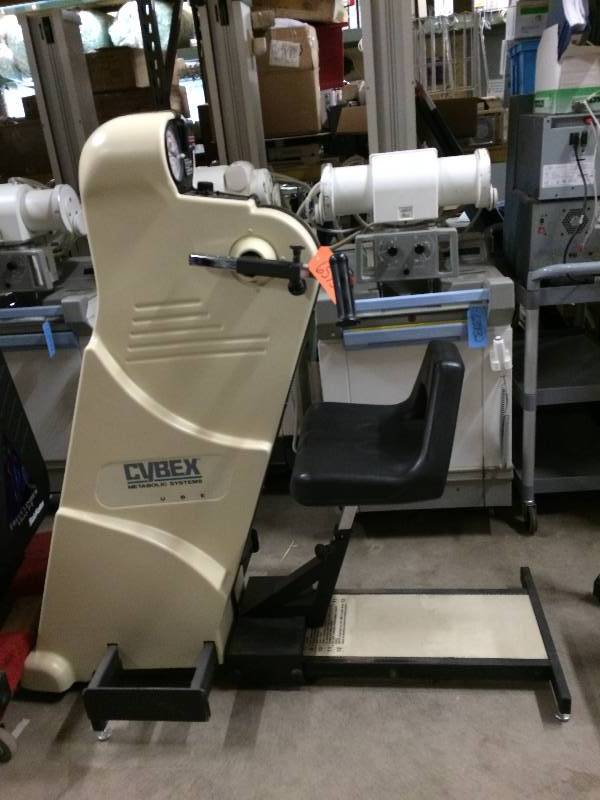The image depicts an industrial-looking setting that resembles a factory or warehouse with concrete floors and steel columns. In the foreground, there is a distinctive piece of equipment that initially appears to be a type of exercise apparatus. It prominently displays the brand name "Cybex" on its side. The machine features a black and beige seat mounted on it, equipped with various controls including a black lever and a dial on the top. Nearby, a large white cylinder can be seen, although it's unclear whether it is part of the machine or just situated next to it. In the background, the photograph shows additional industrial equipment, possibly mounted on carts, hinting at a manufacturing environment.